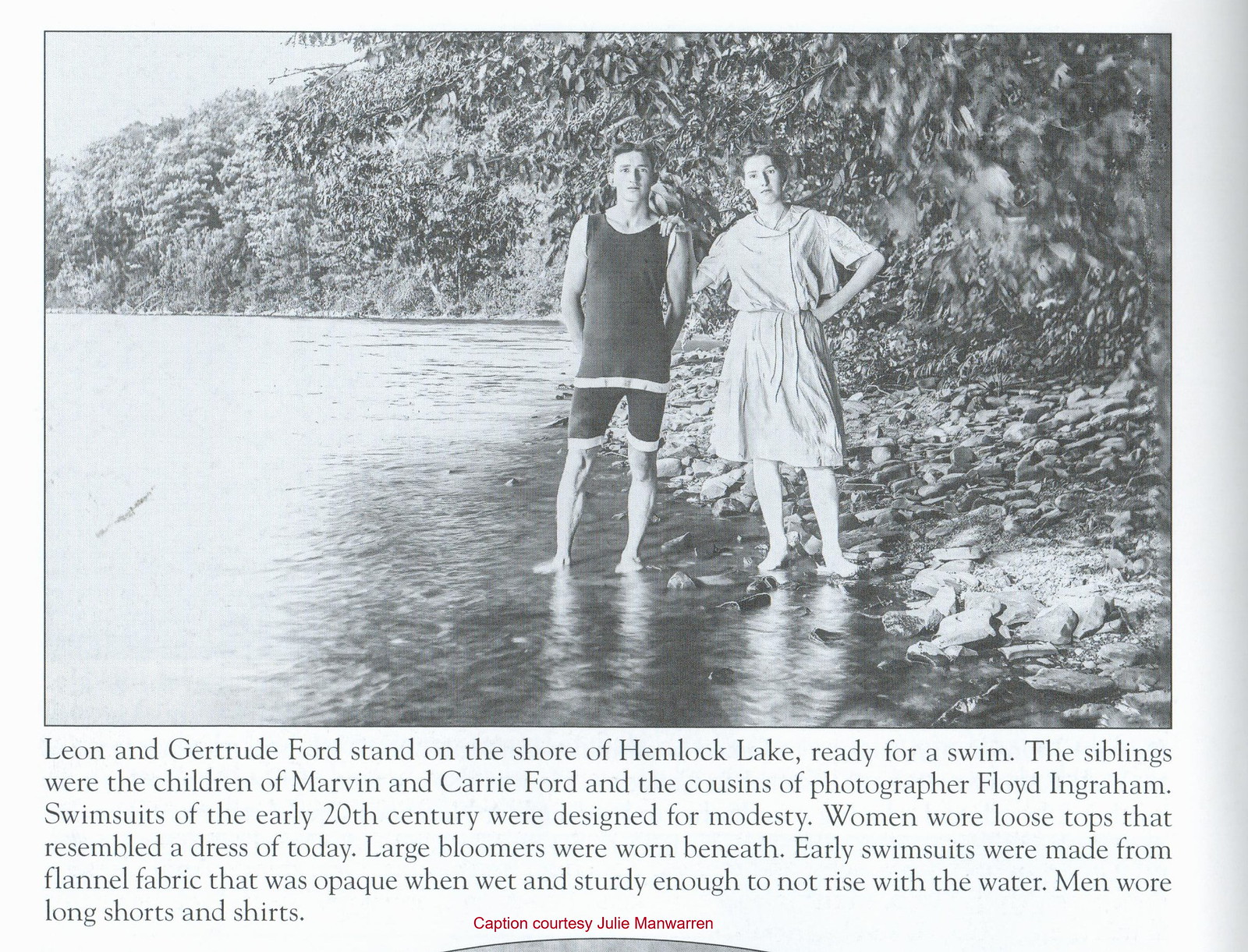This black and white image appears to be a scan of an old book or newspaper article. It shows two people, a man and a woman, standing in foot-deep water at the shore of Hemlock Lake. The man is on the left, and the woman is on the right, both wearing early 20th-century swim uniforms. The shoreline on their right is rocky and lined with many trees, extending far into the background. The caption beneath the image reads: "Leon and Gertrude Ford stand on the shore of Hemlock Lake, ready for a swim. The siblings were the children of Marvin and Carrie Ford and the cousins of photographer Floyd Ingraham. Swimsuits of the early 20th century were designed for modesty; women wore loose tops that resembled dresses of today with large bloomers underneath. Men's swimsuits consisted of long shorts and shirts. Early swimsuits were made from flannel fabric, which was opaque when wet and sturdy enough not to rise with the water. Caption courtesy of Julie Mann Warren."